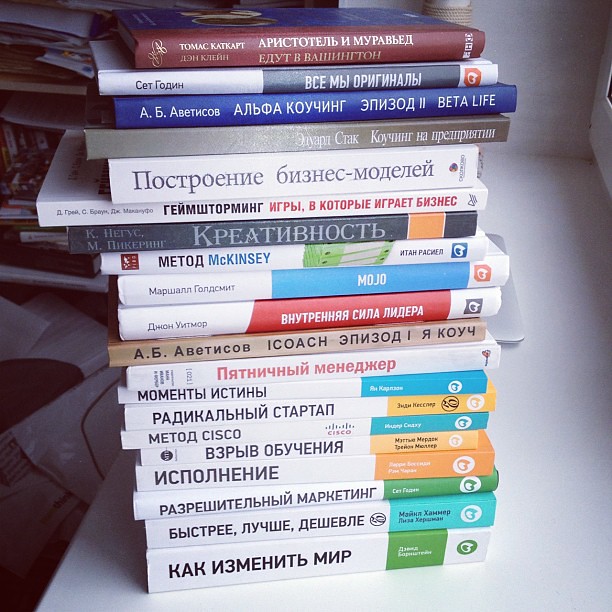This image features a stack of approximately 20 books, neatly piled on a white desk or shelf. The photograph captures the edge of the desk with various items, including additional stacks of papers and a few other books, suggesting a busy, academic environment. The background reveals more shelves with scattered papers, enhancing the academic or work-oriented setting.

The books predominantly feature spines with Cyrillic text, indicating that they are written in Russian or a similar language, though the specific contents remain unreadable. The majority of the books have white spines, with a significant number showcasing uniform logos at the bottom, accompanied by colored stripes in blue, yellow, or green, suggesting a common publisher. Additionally, some books in the stack have spines in red and blue, adding a splash of variety to the mostly white collection.

Overall, this detailed assortment of hardbound and thick paperback books, all with Cyrillic script, presents a visually intriguing and linguistically mysterious scene on a pristine white surface.